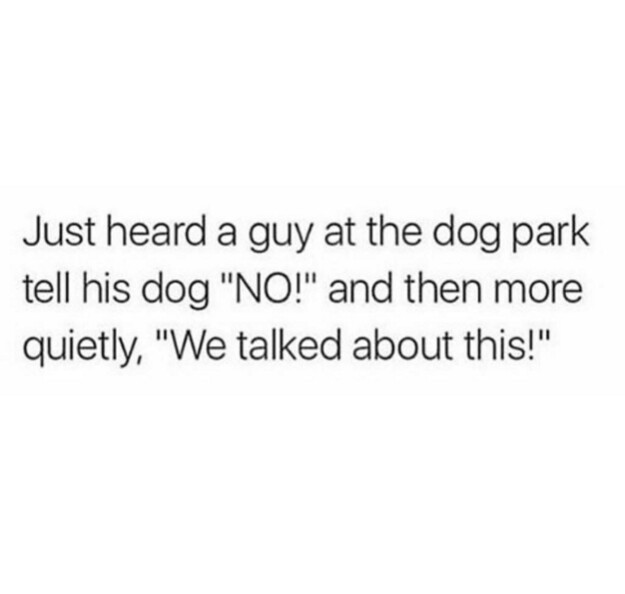An image showcases a humorous quote presented in black font on a white background. The text reads: "Just heard a guy at the dog park tell his dog 'NO!' and then more quietly, 'we talked about this.'" The phrase "NO!" is emphasized in all capital letters with an exclamation point, and both quoted sections add a playful tone to the message. The clean, friendly font is reminiscent of Arial, and there is a faint shadow effect around the words, making the dark gray letters slightly stand out against the white backdrop. Although the image lacks borders or additional graphics, its simplicity accentuates the humor and makes it easily shareable, potentially on social media or quotation sites.